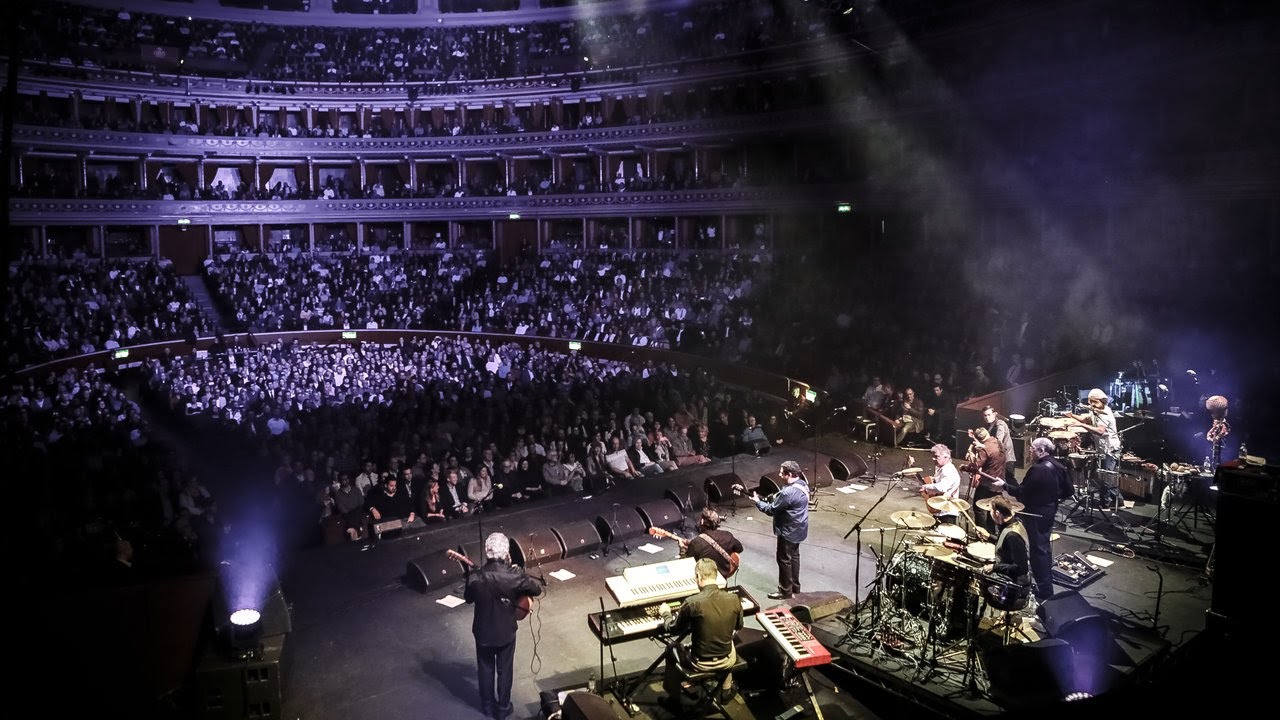This image captures a live concert from a unique perspective behind the stage. The band, composed predominantly of older gentlemen, includes guitarists at the front, a drummer, and a man at a keyboard with both a black and a red instrument, as well as a bassist and someone on bongos. The stage appears somewhat cluttered from this angle. The concert is held in a large, round concert hall that features multiple levels and tiers curving around the venue, including orchestra levels and sky seating. The audience is bathed in a purple-blue light from the stage, filling every level, though details of individual faces and bodies are indistinguishable. The room's architecture and the stage lights, with their accompanying smoke effects, enhance the atmosphere of this vibrant, large-scale event.